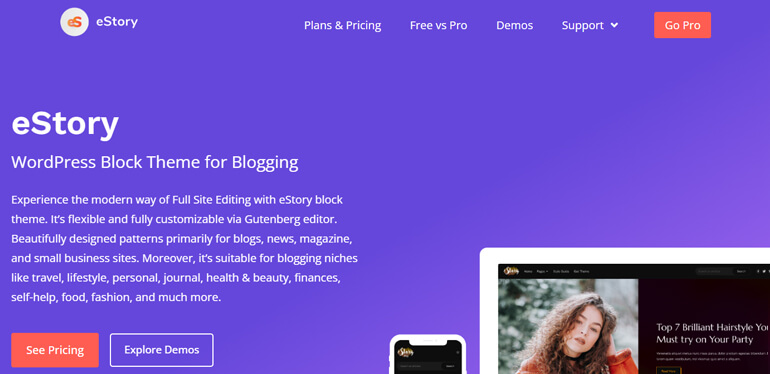This image depicts the homepage of eStory, a company specializing in WordPress themes for blogging. At the top left of the page is the company’s logo. On the top right is a series of links, beginning with "Plans and Pricing," "Free vs Pro," "Demos," "Support" (which features a clickable drop-down menu), and ending with "GoPro," which is highlighted in white within an orange rectangle.

The main body of the website prominently displays the brand name "eStory" and introduces it as a "WordPress block theme for blogging." The text highlights that the theme is flexible and fully customizable through the Gutenberg editor. It describes the design as being ideal for blogs, news outlets, magazine websites, and small business sites. Furthermore, it specifies that eStory is suitable for various blogging niches, including travel, lifestyle, personal journaling, health and beauty, finance, self-help, food, fashion, and more.

In the bottom left corner of the screen, there is an option to "See Prices" and "Explore Demos." The webpage also features an image of a smartphone and a picture of a woman in an orange shirt located at the bottom right corner. This image seems to be indicative of a website or a screenshot of a computer screen, captioned with the heading "Top 7 Brilliant Hairstyles You Must Try at Your Party."